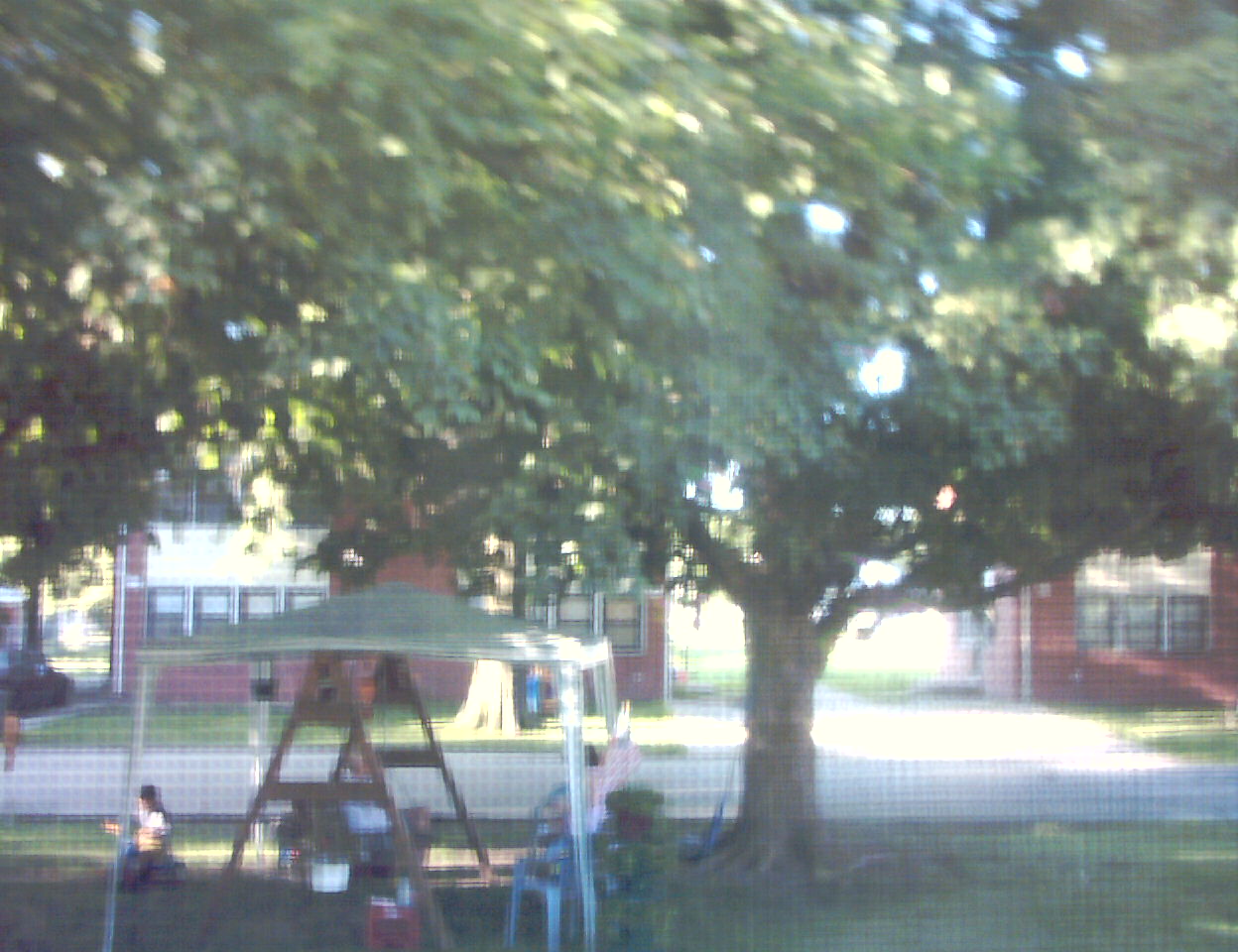The blurry and grainy photograph captures a summertime scene in a residential area, seen through what appears to be a screen door, giving the image a slightly grid-like filter. In the foreground, a public park or yard is visible, surrounded by security wire. The lush greenery features several large, leafy trees providing ample shade, suggesting the season is summer. A man with long, hippie-style hair, reminiscent of the 1970s, is seated under a canopy or gazebo with no sides, supported by wooden stilts. The canopy is topped with a green material, likely intended for shade rather than weather protection. Scattered underneath are plastic picnic chairs and possibly a ladder. Additional elements like a playground set and what appears to be someone playing a guitar add to the scene's leisurely atmosphere. In the background, across a clear road, stand two large red brick houses with many windows, each also boasting well-maintained green lawns.